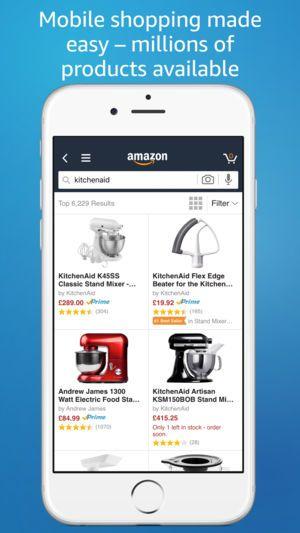The image depicts a website displayed on an iPhone against a blue gradient background that darkens towards the bottom. The website header reads "Mobile Shopping Made Easy, Millions of Products Available," in light blue text. The screen prominently features the Amazon website, where the search term "KitchenAid" has been entered.

On the displayed results, four different KitchenAid products are visible. The first item is the classic KitchenAid Stand Mixer priced at $289. The next item is a KitchenAid Flex Edge Beater, a handheld kitchen tool listed at $19.92. The third product is an Andrew James electric food mixer, which doesn't appear to be a KitchenAid product and shows a non-American price that is unreadable. The final product is a KitchenAid Artisan mixer priced at $152.8.

Additionally, the iPhone's home button is visible at the bottom of the screen, emphasizing that the user is browsing this website on a mobile device. The background's blue color gradient intensifies as it moves downward, providing a visually appealing contrast to the image.